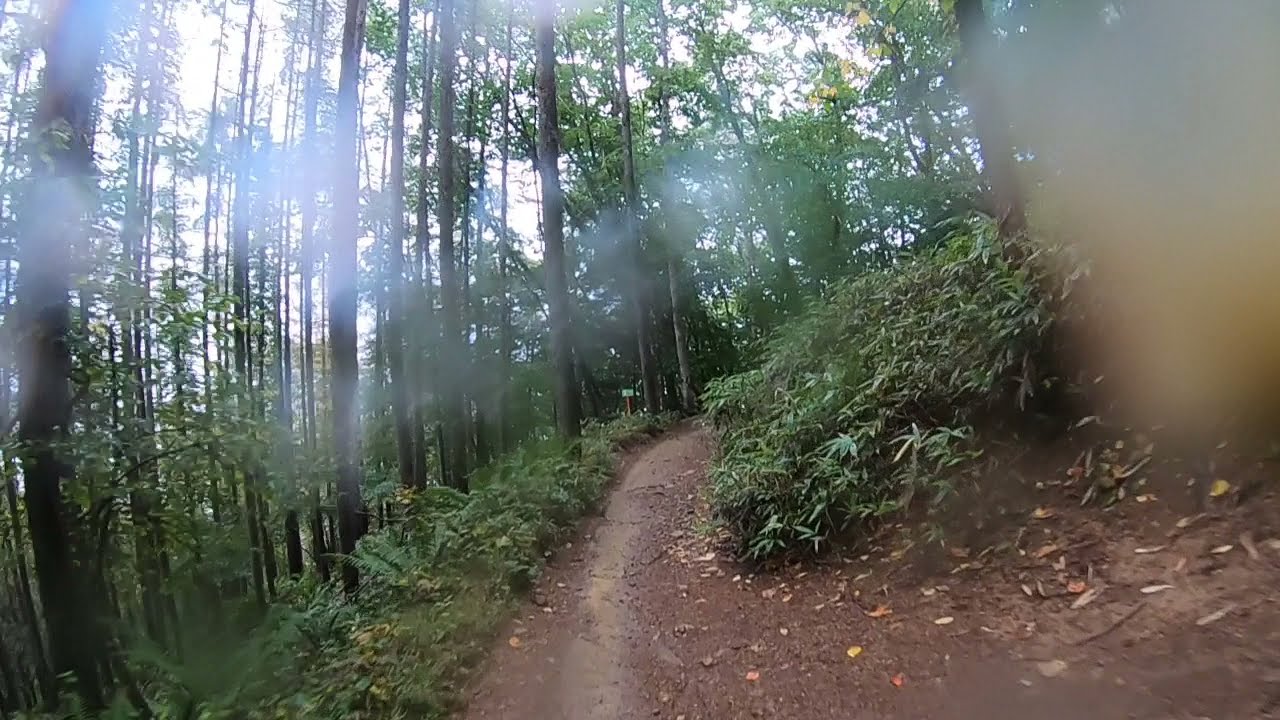In this photograph, you find yourself in a serene forest, gazing upward at a narrow dirt trail that winds uphill and to the right. The forest primarily consists of tall, wide-leaved hardwood trees, with green leaves filtering sunlight and casting a gentle dappled light across the path. A variety of foliage lines the trail, including lush ferns on the left and green bushes, possibly with ivy, wrapping around the slender trees to the right. The ground is a mix of soil, some patches of dead leaves—predominantly yellow and orange—especially visible on the lower right-hand side. Higher up and along the trail, the scene appears somewhat hazy, as if there's a haze of water droplets or smudges on the camera lens, adding a dreamy, ethereal quality to the upper portion of the image. The overall impression is of a sunny yet shaded woodland path, inviting and full of natural detail.